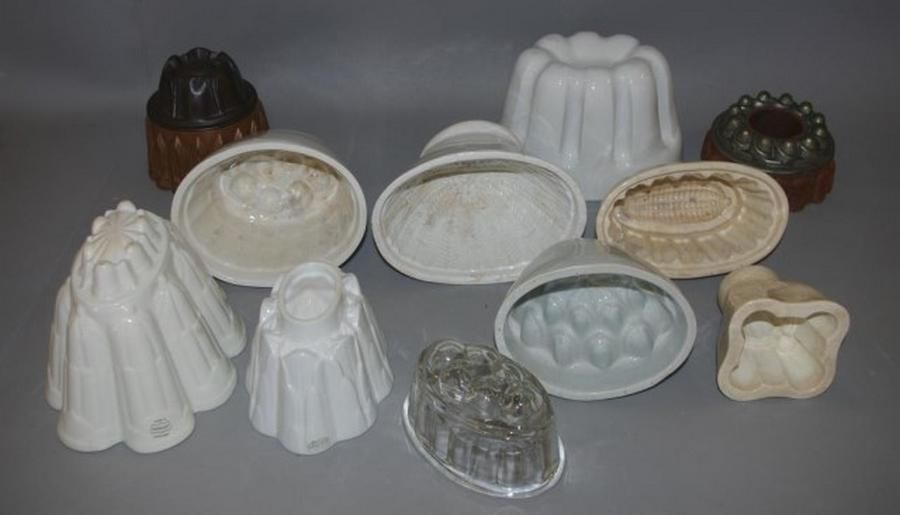The image showcases a diverse collection of different jelly molds arranged in front of a grey background. These molds, primarily designed for creating intricate gelatin shapes, are made from various materials including white porcelain, clear and translucent plastic, and even black and glass-like substances. They feature a range of detailed designs meant to produce decorative shapes for gelatin or other foods. Each mold varies in size and shape, from long and deeply grooved to small and stout. Notable examples include a long, deeply folded mold in the front left, a smaller but similar one next to it, and a clear plastic mold on the right. The back left mold has a knob shape with a large brown base, while the back middle showcases a large, white ceramic jelly mold. The collection evokes a nostalgic feel, reminiscent of traditional molds possibly used for jello, mashed potatoes, or other creative culinary presentations.